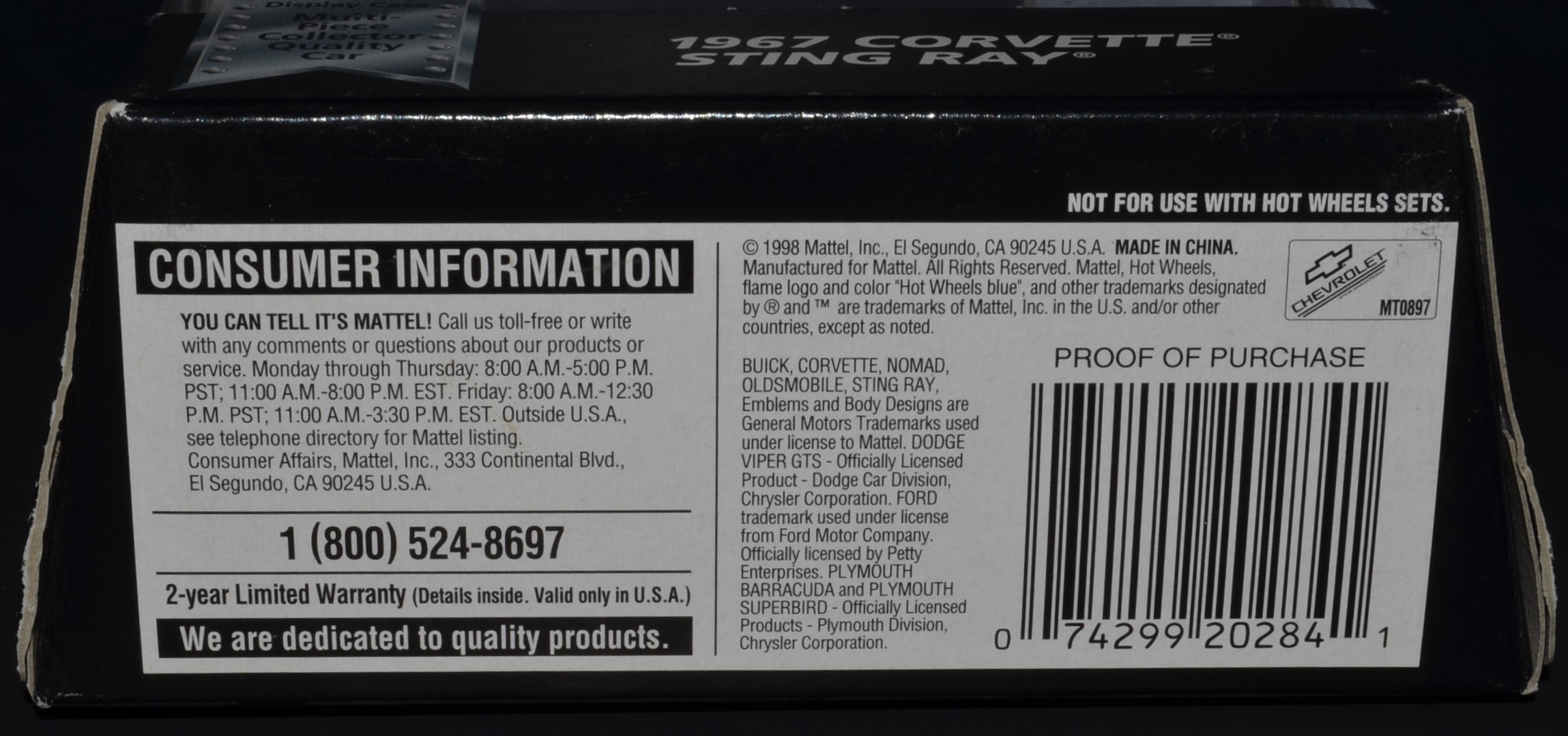The image depicts the back packaging of a Hot Wheels toy car by Mattel, specifically highlighting a 1967 Corvette Stingray model. The side packaging prominently features the text "1967 Corvette Stingray," confirming the car model. The back of the packaging includes a disclaimer stating, "Not for use with Hot Wheels sets," likely indicating that this particular car is sold separately and not intended for use with Hot Wheels tracks. Additional text mentions other car models such as Buick, Corvette Nomad, and Oldsmobile Stingray, along with other consumer information presented on a white panel. Mattel's dedication to quality is emphasized with a message that encourages consumers to call a toll-free number or write with any comments, highlighting a two-year warranty. A barcode and proof of purchase are visible on the right-hand side. The packaging also indicates that the item was manufactured in 1998 by Mattel Incorporated.